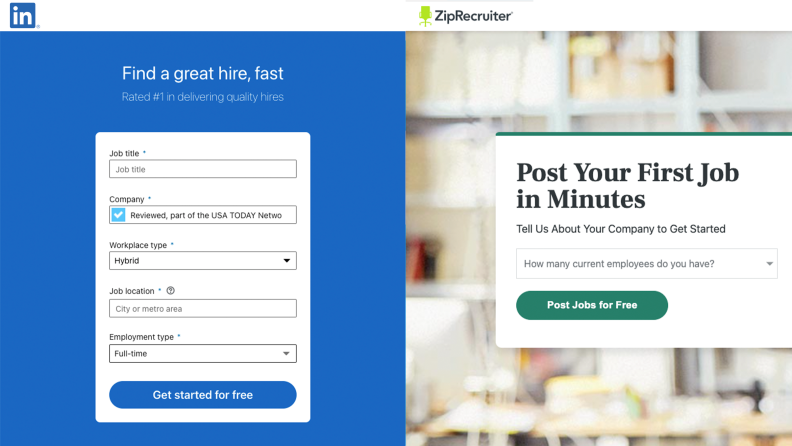This image is a screenshot of the ZipRecruiter home screen. At the top, the ZipRecruiter logo is clearly visible, featuring an office chair icon alongside the company name in black text. The screen is divided into two distinct sections.

On the left side, a blue rectangular box is featured with the bold headline, "Find a Great Hire Fast," followed by the claim, "Rated number one in delivering quality hires." Below this, there are labeled boxes for inputting information, such as "Job Title" and "Company," both accompanied by text boxes for user entry. Also within this section is a statement indicating that the service is reviewed as part of the USA Today Network, denoted by a blue check mark. Further down, there are options to specify "Workplace Type," which is selected as "Hybrid" from a drop-down menu, and "Job Location," where users can input a city or metro area. Additionally, there’s an "Employment Type" drop-down menu with "Full Time" selected. The section concludes with a prominent blue oval button labeled "Get Started for Free."

The right side of the screen depicts a blurred image resembling a home office setup. Over this blurred background is a white box containing the text "Post Your First Job in Minutes," encouraging users to "Tell Us About Your Company to Get Started." Below this prompt, a drop-down menu asks, "How Many Current Employees Do You Have?" Completing this section is a green oval button that says, "Post Jobs for Free."

Overall, the design is clean and organized to guide users efficiently through the process of posting job listings.